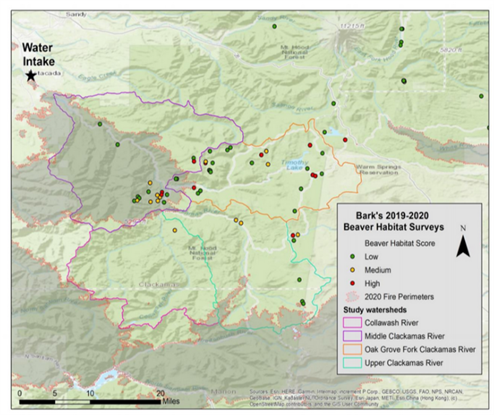The image depicts a detailed geographical map focused on beaver habitat surveys for the years 2019 to 2020. The title "Water Intake" is prominently displayed in black letters in the upper-left corner. The map's surface area is shaded in light green and includes various annotations and geographical features like fire perimeters and watersheds, marked by different colored lines. 

In the lower-right corner, a white rectangle serves as the legend, explaining the color-coded beaver habitat scores. The survey results are represented by dots in three colors: green for low occupancy, yellow for medium occupancy, and red for high occupancy. Most dots are green, indicating predominantly low beaver occupancy, with fewer yellow and red dots scattered near streams and lakes signifying medium and high occupancy, respectively. The map also includes areas of interest marked with beige-colored key legends.